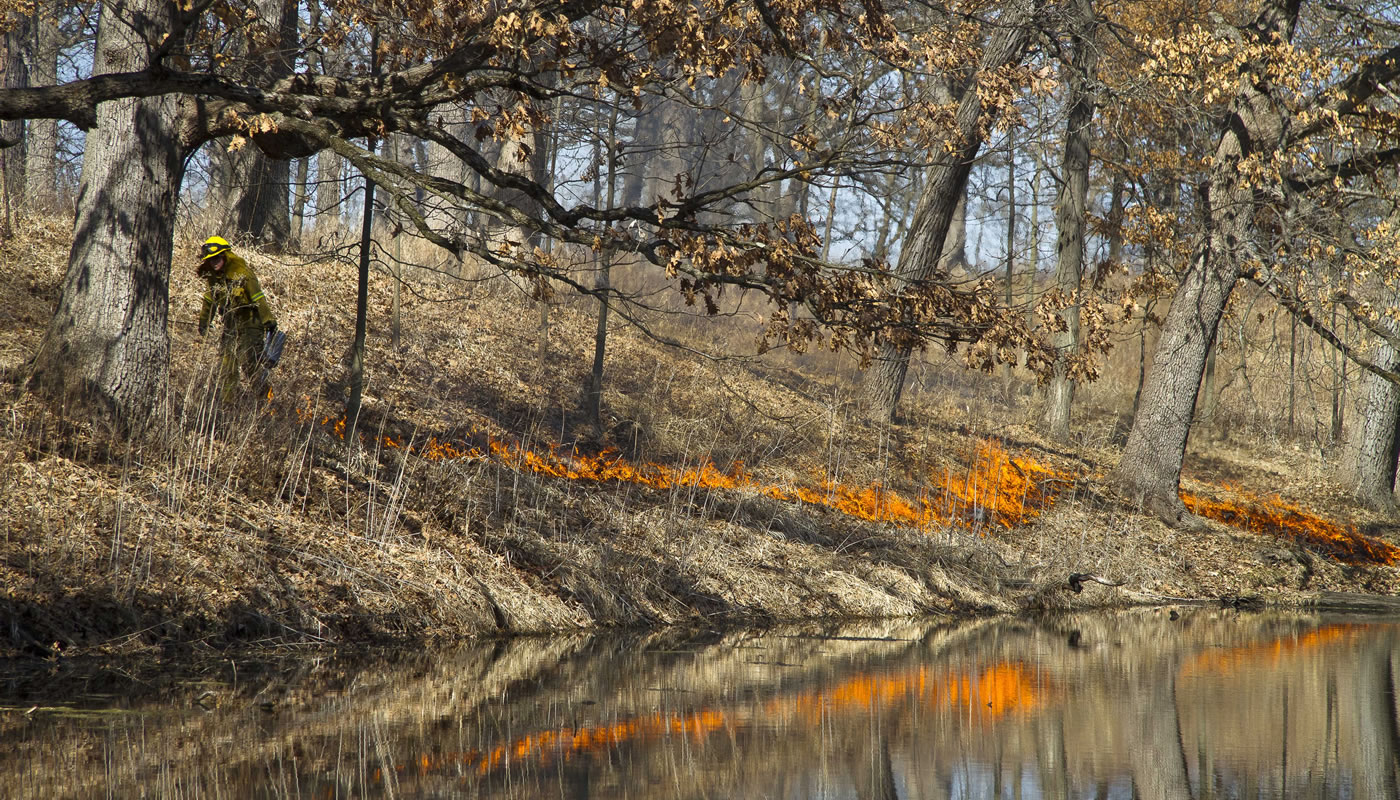This photograph captures a striking scene of a forest affected by a controlled brush fire. In the foreground, there's a body of water that reflects the flames and the barren trees. The central focus is a line of fire snaking through the dead grass and fallen leaves, hinting at a deliberate burn. The trees are varied in size; larger ones are on the left and smaller ones are scattered towards the center and right, with most leaves turned brown or fallen, indicative of fall. On the left side, a fireman in full gear—including a yellow jacket and helmet—carries a gas can, contributing to the managed burn. The background shows a morning sky through the stark, leafless branches. The forest appears lifeless, and the scene is solemn yet organized, reflecting both the desolation of fall and the precision of controlled forest management.